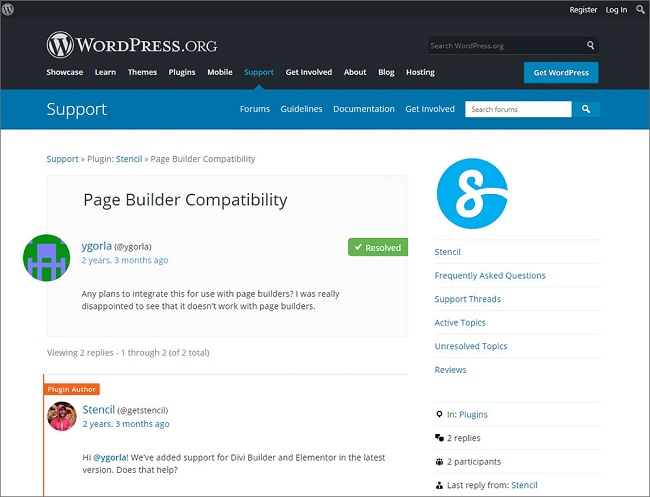The image displays the support page for WordPress.org, featuring a well-organized layout with a black navigation bar at the top. This navigation bar includes clickable sections such as Showcase, Learn, Themes, Plugins, Mobile, Support (highlighted in blue), Get Involved, About, Blog, and Hosting. To the right, there's a prominent blue button labeled "Get WordPress" and a black search bar reading "Search WordPress.org." In the upper right corner, the options to Register and Login are visible.

Below the navigation bar, a secondary blue support bar offers additional options: Forums, Guidelines, Documentation, and Get Involved, along with another search bar accompanied by a blue search button.

The main content area highlights a forum post regarding "page builder compatibility." The post, written by a user named YG Orla two years and three months ago, expresses disappointment over the lack of page builder support. Adjacent to the post, a green "Resolved" button with a checkmark indicates that the issue has been addressed. The post shows two replies, with the first from the plugin author, "Stencil," stating that support for DV Builder and Elementor has been added in the latest version, replying two years and three months ago.

On the right side of the page, there's a section with a distinctive "G" logo and information about "Stencil," including frequency of questions, support threads, active topics, unresolved topics, reviews, location in plugins, two replies, two participants, and the last reply from Stencil. This support page exemplifies WordPress.org's commitment to providing timely and helpful responses to its users' technical questions.